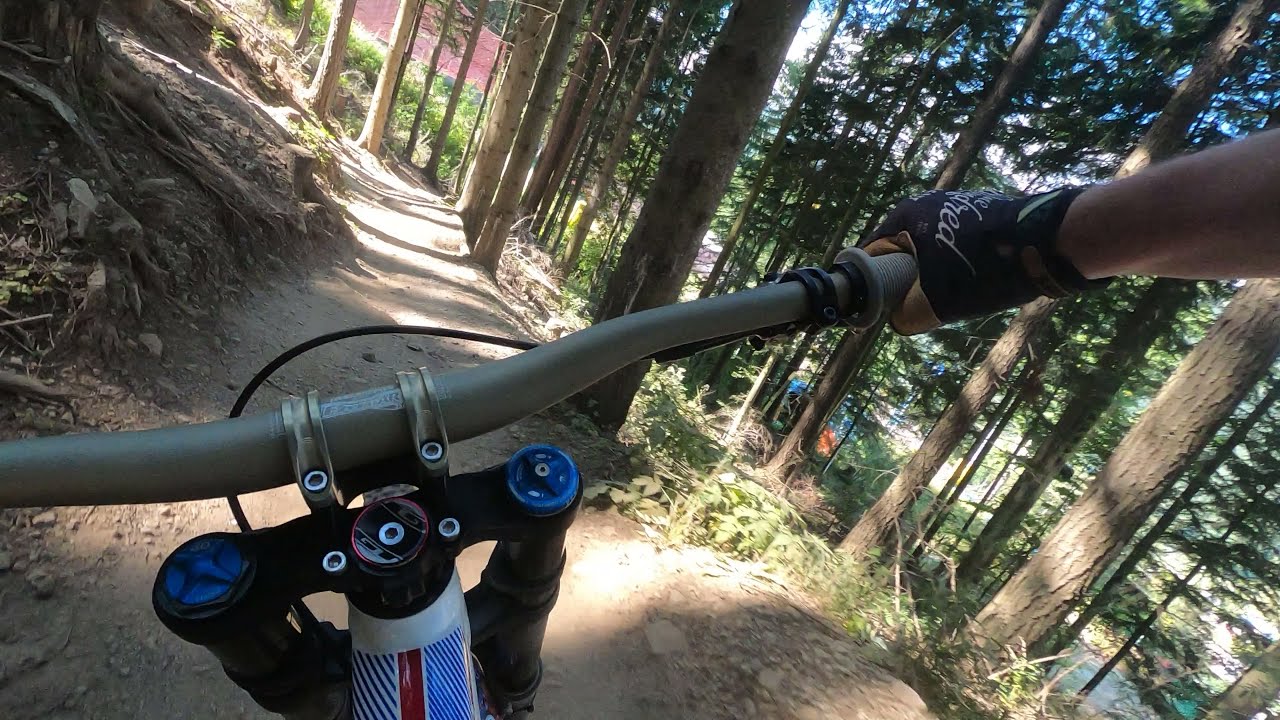The image captures the perspective of a rider navigating a dirt mountain trail through a dense forest in broad daylight. The light-colored dirt trail winds from the center of the image slightly towards the left and is intersected by shadows cast by towering pine trees on the right side, with patches of sky and clouds visible through their green needles. The trail appears smooth but has rocks lining its edges and large tree roots emerging from the left.

Visible from the rider's viewpoint, the handlebars of the bicycle are a light gray color, held in place by silver bolts, with a slight curve at the center. A black cable for the brakes runs through the middle of the handlebars. Only part of the bicycle frame is visible; it is predominantly red with diagonal blue stripes, while the arms extending down to the tires are black.

A gloved Caucasian hand, covered in a black glove with cream-colored sections on the palm and underside of the fingers, grips the right side of the handlebars. The rider's forearm extends from the top right corner of the image. In the distance, peeking through the trees, there is a glimpse of what appears to be the red roof of a building, adding a pop of color against the natural greens and browns of the forest.